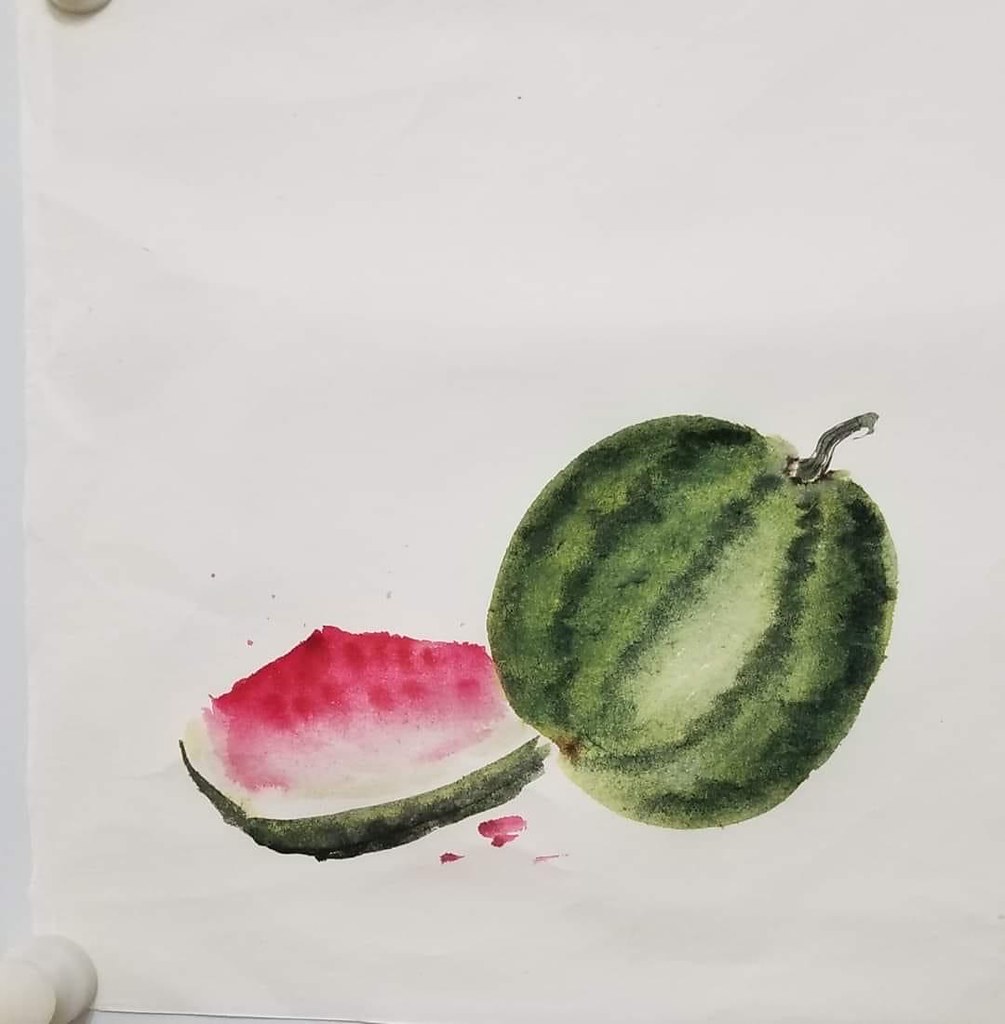Displayed on a white wall, this detailed painting or drawing is securely held in place by a white pushpin located in the bottom left-hand corner. The artwork features two watermelons: one whole, uncut watermelon and one quartered piece. The whole watermelon, prominently showing a stem at the top, suggests it has recently been plucked from a vine. The cut section vividly captures the juicy, red flesh, bordered by a white rind and enveloped in a green skin, highlighting the watermelon’s freshness and ripeness.